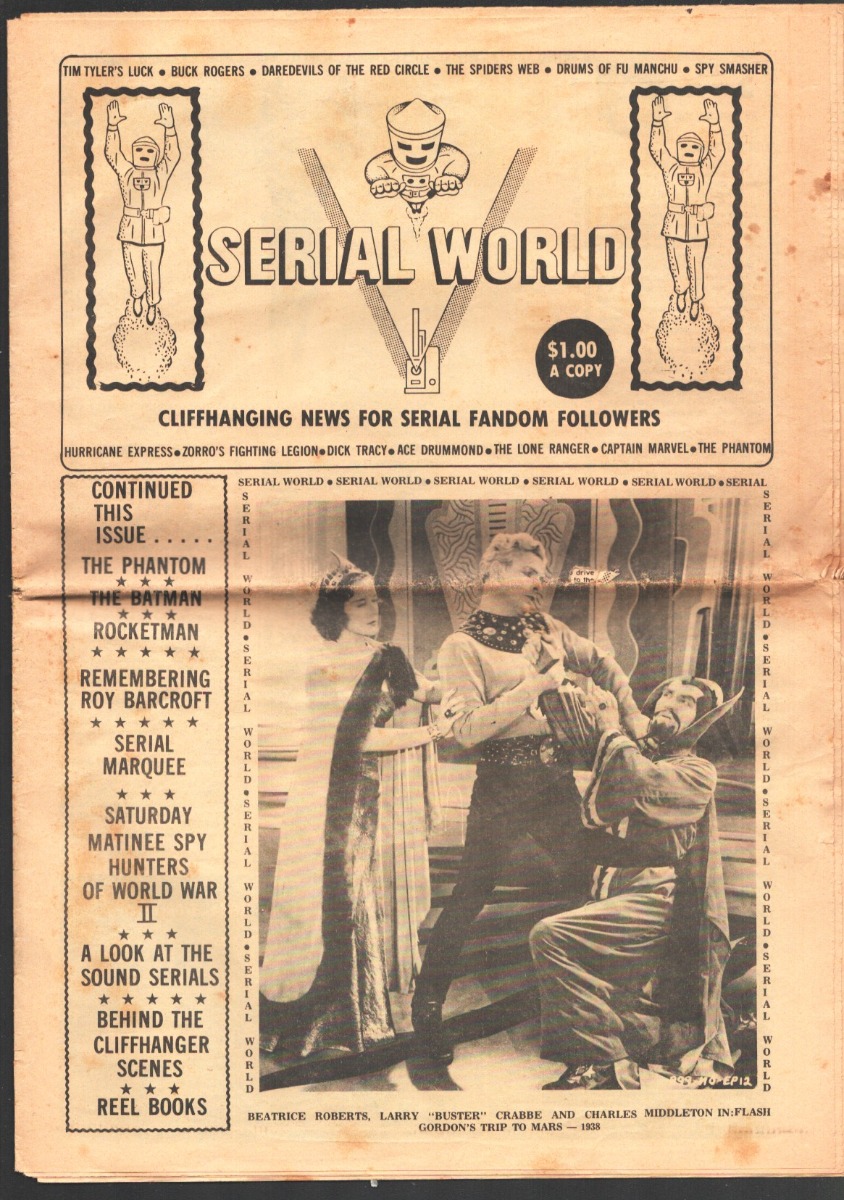The image is an advertisement, presumably from an old black and white newspaper or pamphlet, titled "Serial World". At the top, "Serial World" is flanked by identical images of a man standing on a ball with both arms raised skywards, accompanied by an illustration of a man flying towards the viewer with outstretched arms. This promotional material, priced at $1 a copy, offers "cliffhanging news for serial fandom followers."

Below the heading, the ad features a photograph with three characters, suggesting they might be in a play or a serial scene. The central figure, dressed in a Western-style outfit, is engaged in a dramatic confrontation with a wizard-like figure to his right, characterized by a spiky-collared robe and an unusual goatee. To his left, a concerned woman in a long white dress trimmed with black fur and wearing a crown clutches him.

On the left side of the ad, text lists various serials and features, including "Hurricane Express, Zorro's Fighting Legion, Dick Tracy, Ace Drummond, The Lone Ranger, Captain Marvel, and The Phantom," followed by "Continued this issue: The Phantom, The Batman, and Rocket Man; Remembering Roy Barcroft; Serial Marquee; Saturday Matinee; Spy Hunters of World War II; A Look at the Sound Serials; Behind the Cliffhanger Scenes; Real Books." The entire layout is on a yellowed piece of old paper, adding to its vintage appeal.